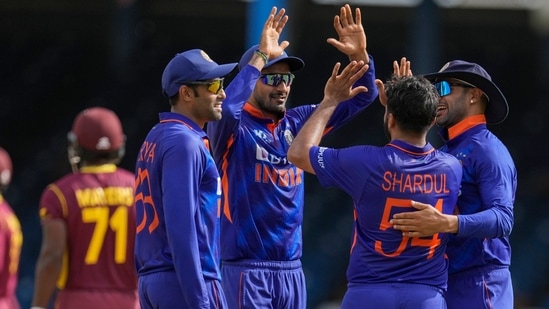This outdoor photograph, taken during the daytime, features a close-up view of four male athletes dressed in coordinated, royal blue uniforms with orange lettering and numbers. Three of the men are wearing long-sleeved shirts, while one is in short sleeves, and all have matching blue shorts or pants. The frontmost athlete’s shirt reads "Shardul" with the number 54 in prominent orange letters. In this scene, two athletes have blue baseball caps, one a dark blue safari-style hat, and one is hatless. They are grouped in a circle, facing each other, with joyful expressions. One of Shardul’s teammates has his arm around his back, while two of the men are poised to exchange high-fives, both donning sunglasses. The background is blurred, hinting that they are likely outside, with hints of maroon-clad opponents, probably the opposite team, visible in the distance. One blurred figure in the back, wearing a maroon outfit with yellow lettering and a maroon cap, bears the number 71 and has short sleeves, distinguishing them from the main group.